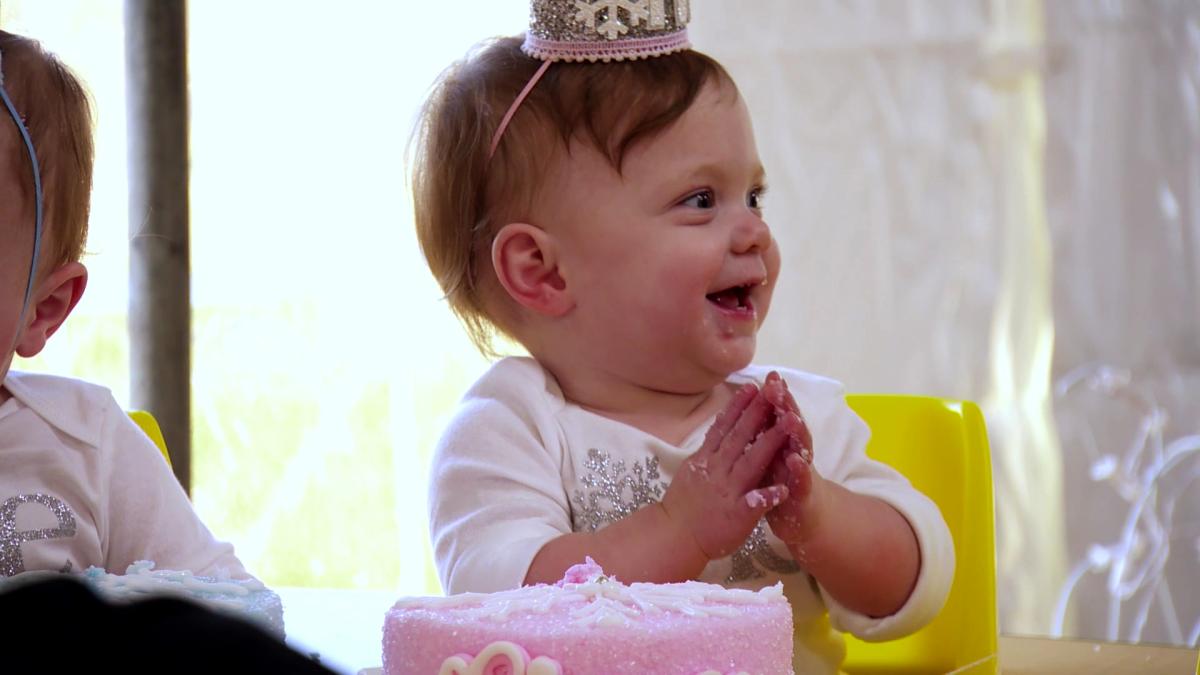A cheerful one-year-old girl celebrates her first birthday. She sports a sparkly birthday hat with a pink band, positioned adorably on her short brown hair. Her big brown eyes gleam with excitement as she looks up to the left, her tiny nose and wide, open-mouthed smile adding to her infectious joy. She sits in a yellow plastic chair, dressed in a white shirt with rolled-up sleeves. Her hands, covered in frosting, are clasped together as if in a prayer pose. In front of her is a pink birthday cake, evidently touched and explored thoroughly by the birthday girl. This enchanting scene captures the pure delight of a child's first milestone celebration.